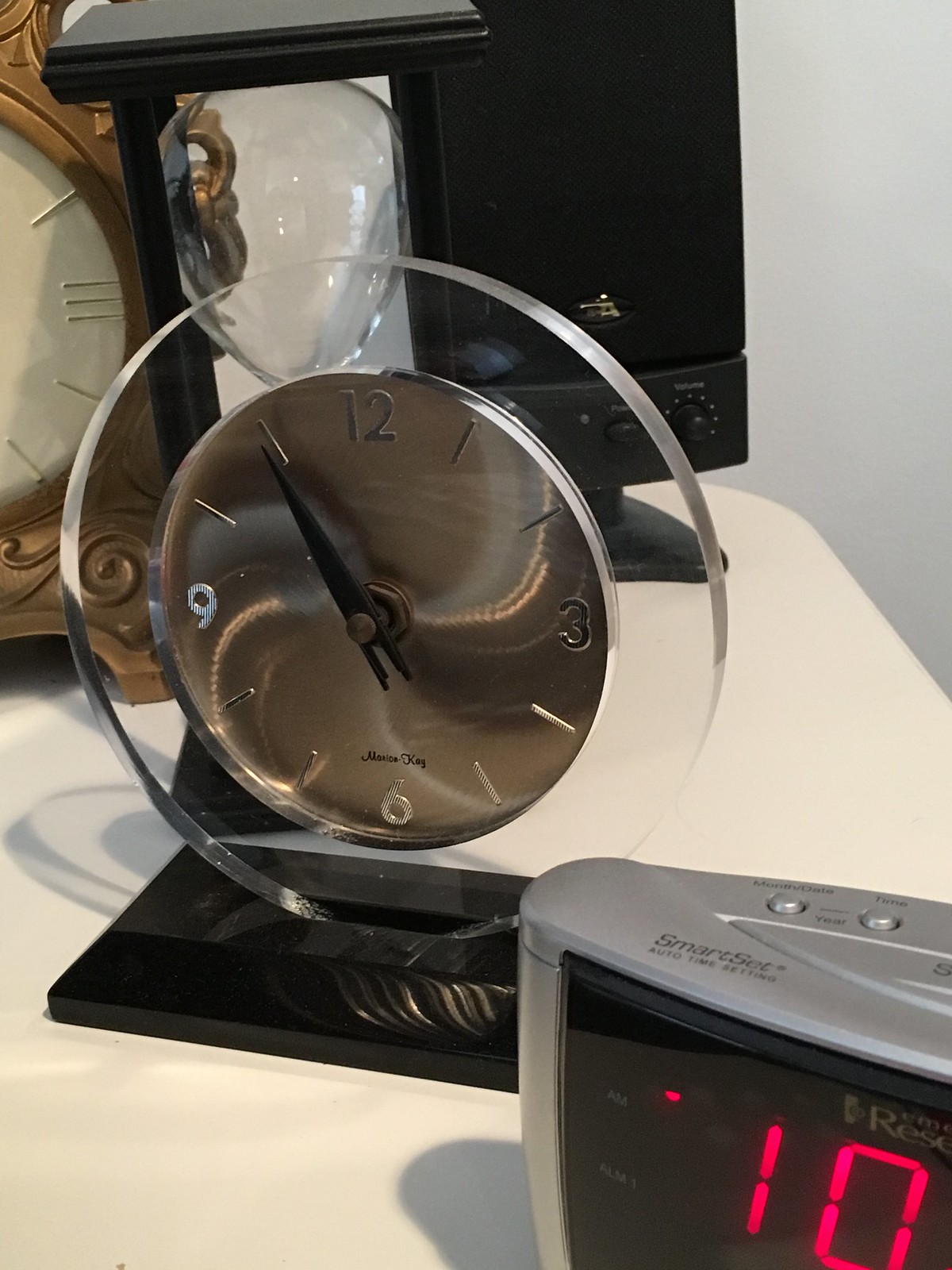The image showcases a variety of clocks poised on a pristine white table. In the right foreground, there is a partially visible digital alarm clock with a gray body and a black screen, displaying the numbers '10:10'. Only about 20% to 25% of this clock is in view. 

To the left of the digital clock, positioned centrally in the image, stands a round pedestal-style clock. This clock features a clear, glass-like outer casing with a black pedestal base. The clock face itself is silver, with muted silver numbers, creating a sleek and understated look. The edges of this clock are transparent, adding an element of depth.

Behind the pedestal clock, the top half of an hourglass encased in a brown wooden frame is noticeable, hinting at the passage of time. To its right, a black speaker with various knobs and dials is visible, adding a modern touch to the assortment.

In the upper left corner of the image, only about 20% of a brass clock can be seen. This clock has a white face, providing a classic contrast to the other timepieces displayed. The variety of styles, from digital to antique, illustrates a broad timeline of timekeeping devices.